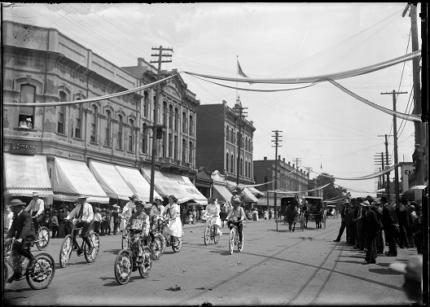This detailed black-and-white photograph from the early 20th century, possibly around the 1910s or 1920s, captures a lively scene in a prosperous town or small city. The image, bordered by black lines, showcases a bustling street lined with multi-storied buildings of British architectural influence, characterized by royal patterns and designs, with shops on the ground level covered by light-colored awnings. 

A significant number of people are gathered, hinting at a celebration, perhaps the end of World War One or an Independence Day parade, as decorations on the bicycles suggest a patriotic theme with red, white, and blue elements. The crowd includes men in light shirts, dark ties, pants, and hats, and women in light dresses, some of whom are riding bicycles. There's also a mix of horse-drawn buggies in the background, indicating the coexistence of old and newer forms of transportation.

On the right side of the street, near the sidewalk, a group of people has congregated, likely spectators watching the cyclists. The street itself appears clean and organized, with visible electrical poles and wires, hinting at modern amenities for its time. Streetlights and lampposts are also present, bathing the scene in daytime sunlight, evidenced by the bright sky and illuminated ground.